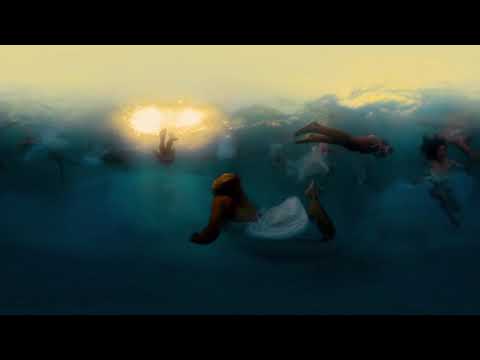This enchanting painting depicts an underwater scene filled with whimsical and fantastical elements. Dominated by shades of blue and green, the scene showcases multiple fully clothed swimmers, creating a dreamlike atmosphere. On the left, dark figures disappear into the depths, while on the right, three swimmers are caught in various swimming poses. A prominent figure in a red shirt and white pants, or possibly a dress, stands out as they swim to the right. Amidst the underwater scene, a bright yellow area at the top middle suggests someone falling into the water. Above the aquatic tableau, light yellow and gold clouds stretch across a sky that transitions from blue to darker hues, adding to the surreal quality. The water itself appears darker as it deepens. The overall effect of the painting is both whimsical and fantastical, suggesting a magical world under the waves.